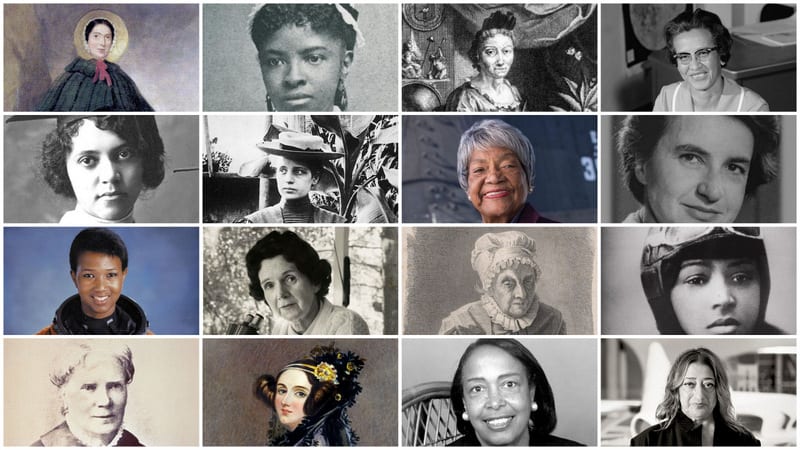This is a collection of 16 photos of women from various historical periods, showcasing both black and white and colored images. The first image in the upper left depicts a woman in a long black robe with a red string around her neck and a yellow wide-brimmed hat, appearing to be either white or possibly Asian. Next to her is a black-and-white photo of a young black girl with white ribbons in her hair. The third image is a black-and-white drawing of an elderly woman with a mid-cut top and a dragon statue behind her. The fourth image shows a smiling woman in black and white, wearing a shirt with a white stripe. The fifth is another black-and-white image of a girl with dark curly hair. The sixth photo is a woman in a brimmed hat like Mary Poppins, holding a plant. The seventh is a recent picture in color of an older black woman with short gray hair, smiling. The eighth is a black-and-white close-up of a woman's face. The ninth shows a black woman in what appears to be an astronaut suit. The tenth is a black-and-white picture of an old lady with dark curly hair. The eleventh is a sketch of an older woman with a lumpy white hat and a white collar. The twelfth is a black-and-white photo of a pilot woman, showing only her face. The thirteenth is another sketch of an older woman with two buns in her hair. The fourteenth image is a drawing of a woman with fancy dark brown hair and a golden decoration. The fifteenth is a black-and-white photo of a black woman with earrings and straight hair. The sixteenth, and final, picture is a black-and-white image of a woman with lighter hair and a dark jacket, showing a serious expression. This diverse array of women, spanning from the 1800s to modern days, suggests they were all influential figures in history.